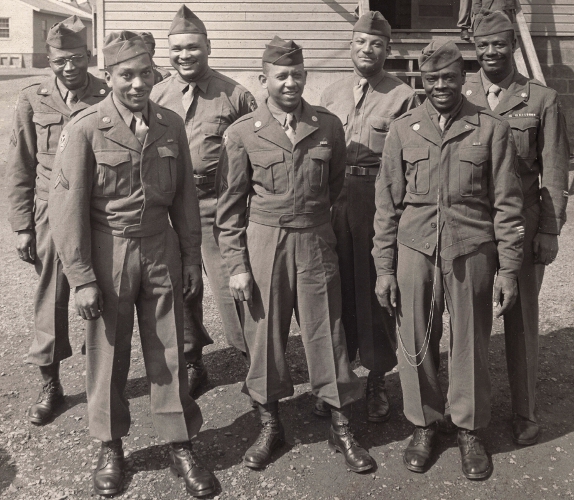This sepia-toned black-and-white photograph depicts seven young black military service members from the World War II era, standing in front of a barracks-style building with siding and steps leading up to an open door. Arranged in two rows, with three men in the front and four in the back, the men are posed and smiling, likely for a photo to send home. They are all wearing military uniforms, which include buttoned jackets with collars and lapels, dress shirts with ties, dress pants, and black leather boots. Some of the men sport patches on their sleeves and various pins, with one man in the back row displaying a row of medals on his chest. Interestingly, while all are outfitted in military attire, three men in the front are dressed in fatigues, whereas those in the back are in formal uniform with overcoats topped by peaked caps. The ground they stand on is mostly dirt with scattered gravel.